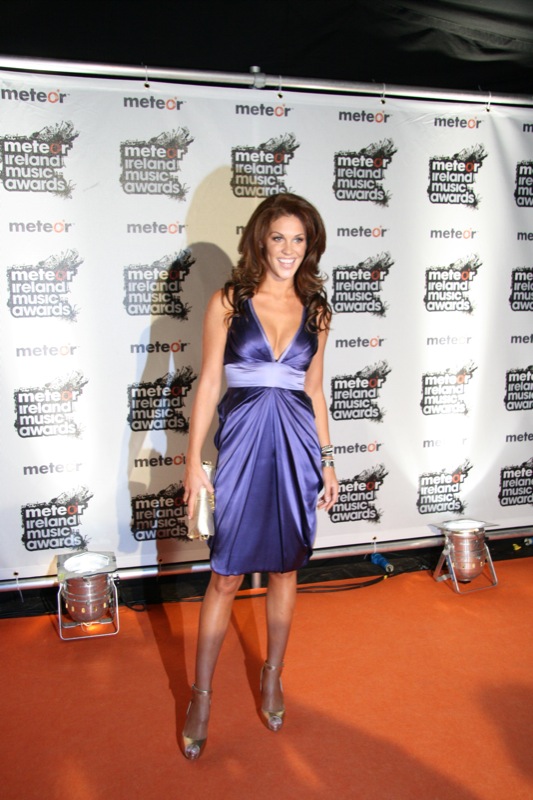A tall brunette woman with shoulder-length, long curly hair is posing on an orange carpet at a red carpet event. She is wearing a mini gown that features a deep V-neckline and varies in color from purplish-blue to blue. The waist of the dress is a lighter shade of blue. She accessorizes her look with a metal bracelet on her left wrist and a golden clutch in her right hand. She is also wearing silver shoes. Her cleavage is visible, and she is smiling brightly at the camera. Behind her, a large white banner is displayed with the words "Meteor Island Music Awards" repeatedly printed on it. The banner is illuminated by flashlights, giving prominence to the event's name.